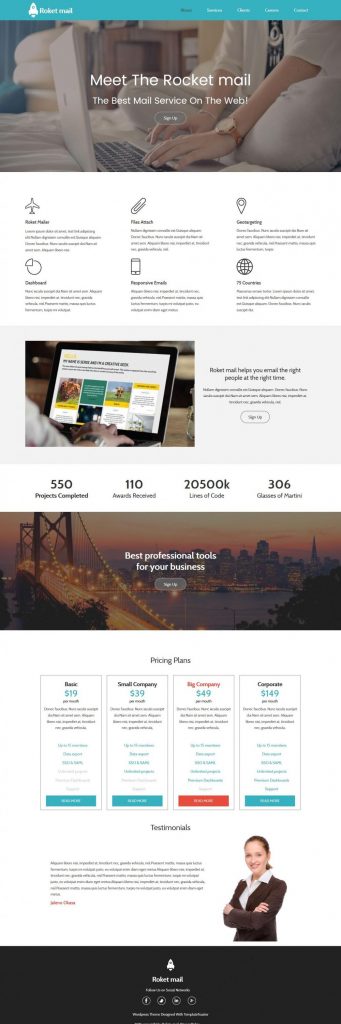### Advertisement for Rocket Mail Email System

At the top of the page, there's a green notification bar featuring a bell icon and the text "Rocket Mail". The menu includes six items, with "Home" being highlighted to indicate the current page.

The main content is divided into six distinct sections:

1. **Introduction**: A large heading reads "Meet Rocket Mail, the Best Mail Services on the Web". This section includes a graphic depicting a person sitting cross-legged on a bed, typing on a laptop, symbolizing convenience and user-friendliness.

2. **Features**: A white section that appears to list the key features of Rocket Mail, although not all details are clear. Icons include an airplane (likely signifying fast mail delivery) and a paperclip (probably referencing attachment capabilities).

3. **User Interface**: Shows another person working on a laptop. This part seems to display detailed metrics such as the number of lines of code (20,000) and other mysterious figures (550 something and 110 something).

4. **Business Tools**: This section contains a photo in the background, possibly of a well-known bridge. The text advocates renting professional tools for business purposes.

5. **Pricing**: Details different pricing plans, providing potential customers with options according to their needs.

6. **Contact Information**: Features a photo of a consultant with folded hands, indicating that customer support is available for inquiries.

This thorough and structured layout emphasizes Rocket Mail's capabilities, user benefits, and support features, making it an appealing choice for potential users.